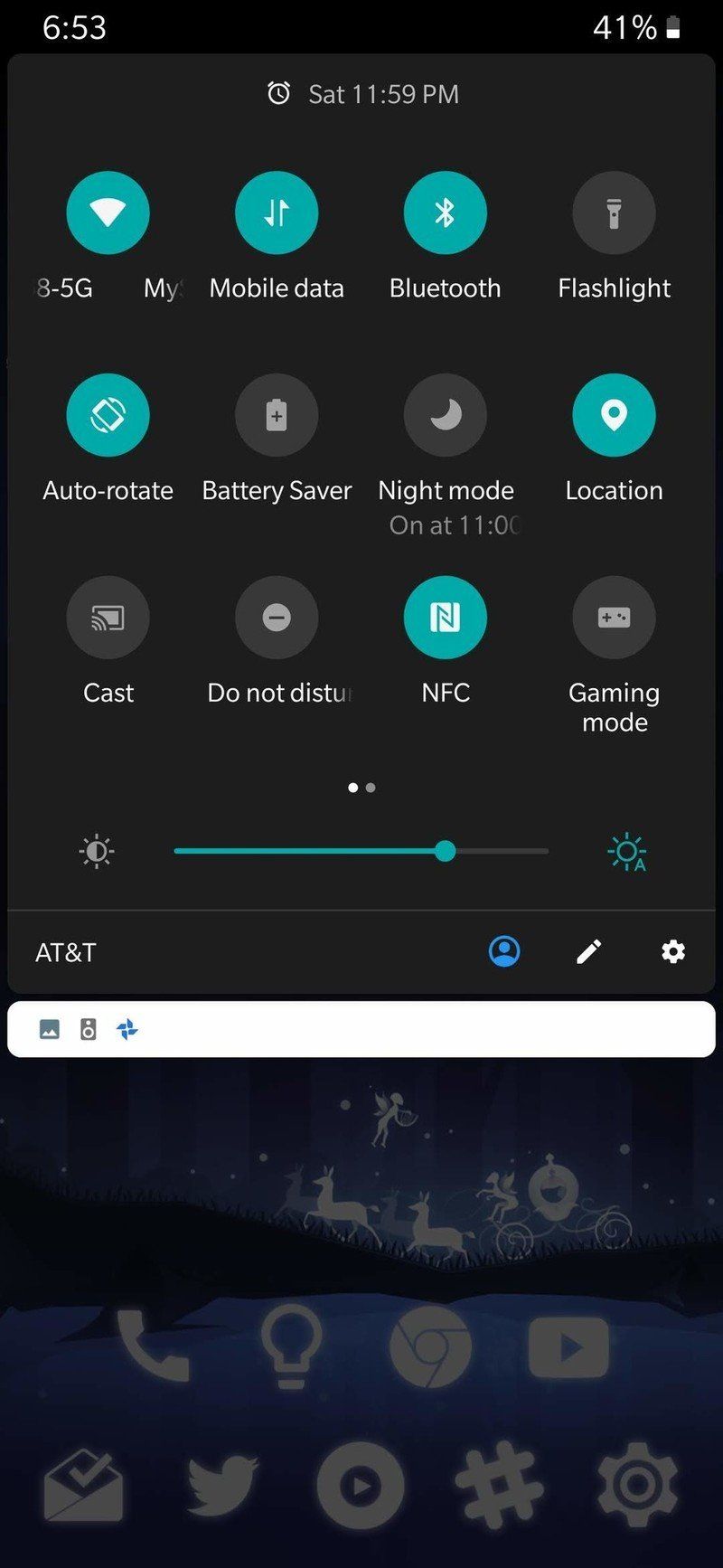The image depicts a smartphone settings screen with twelve icons arranged in three rows of four. The icons in each row represent various phone settings, some of which are highlighted in blue indicating they are active, and others are gray, indicating they are currently deactivated.

### Top Row:
1. **Wi-Fi** - This icon, which shows signal strength bars, is highlighted in blue, indicating that Wi-Fi is turned on.
2. **Mobile Data** - This icon is also highlighted in blue, showing that mobile data is active.
3. **Bluetooth** - Highlighted in blue, indicating Bluetooth is enabled.
4. **Flashlight** - This icon is grayed out, indicating the flashlight is off.

### Second Row:
1. **Auto-Rotate** - The icon for this setting is highlighted in blue, indicating that auto-rotate is turned on.
2. **Battery Saver** - This icon is grayed out, showing that the battery saver mode is off.
3. **Night Mode** - Grayed out icon with a note indicating it will activate at 11 PM.
4. **Location** - This setting's icon is highlighted in blue, showing location services are enabled.

### Third Row:
1. **Cast** - The icon for screen casting is grayed out, meaning this feature is off.
2. **Do Not Disturb** - This icon is also grayed out, indicating the feature is not active.
3. **NFC (Near Field Communication)** - Highlighted in blue, showing that NFC is enabled.
4. **Gaming Mode** - This icon, which shows a gamepad controller, is grayed out, indicating gaming mode is off.

At the bottom of these rows, there are two dots: one white and one gray, indicating the currently viewed settings page. Below this indicator is a brightness slider set to approximately 75% of its maximum level. Further down, there is the AT&T service provider name, accompanied by three additional icons: a blue-highlighted user avatar, a white pencil icon for editing, and a white gear icon for accessing general settings.